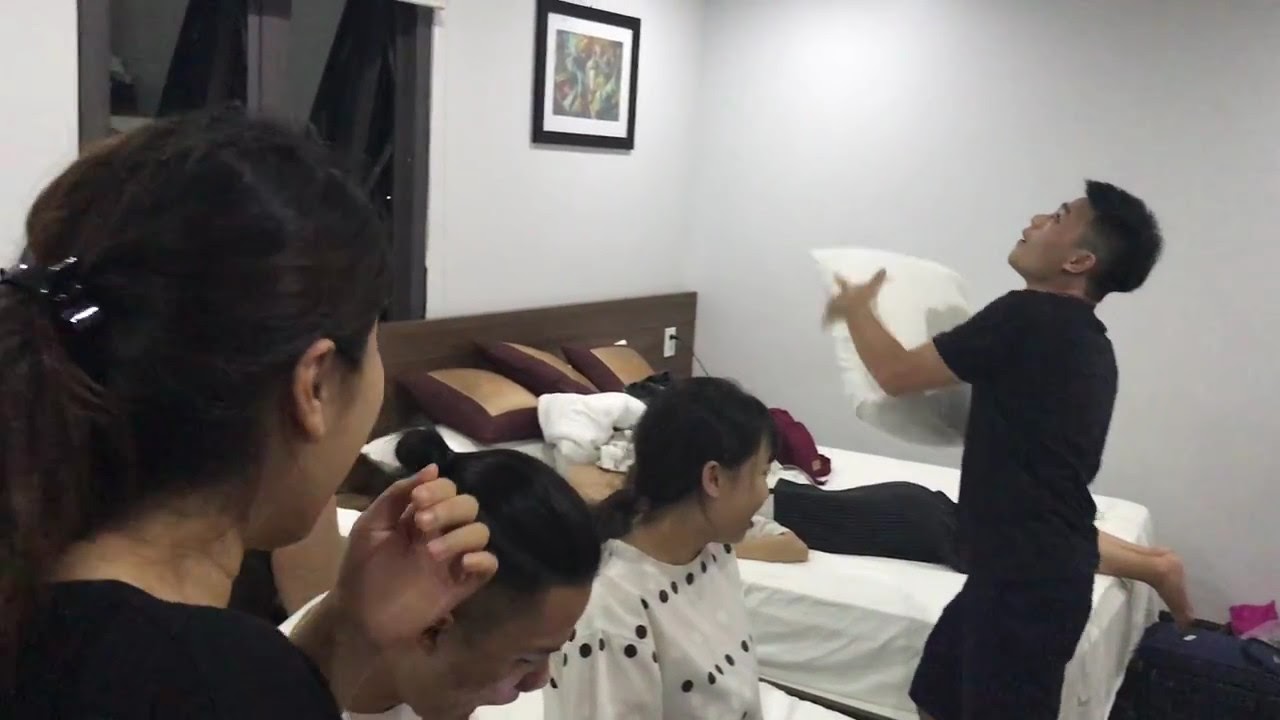The image captures a lively scene in a hotel room or bedroom with white walls and two white beds in the bottom left corner. There are five people in total, engaging in what seems to be playful interaction. Starting from the left, a woman with her hair tied back and her hand raised to her face is seen looking towards the right. Next to her, a man with his hair in a bun is looking downwards. To his right is a woman in a white shirt with black polka dots, laughing as she looks towards the boy on the far right. This boy, dressed entirely in black, is holding a white pillow and looking up, possibly in mid-motion as his hands appear slightly blurry. Behind him, another person lies on the bed with white sheets and pillows, adorned with burgundy and gold cushions. The person on the bed wears black and grey attire, with their feet hanging off the edge. Above the bed, a picture in a black frame with a white border is mounted on the wall, accompanied by a brown wooden headboard. The room also features a possible mirror or window, detailed with black lines. Both beds are neatly made with white sheets, and a few items like hoodies or blankets are scattered on them, adding to the casual, comfortable atmosphere of the scene. No text is visible in the image, and the floor appears to be dark in color.